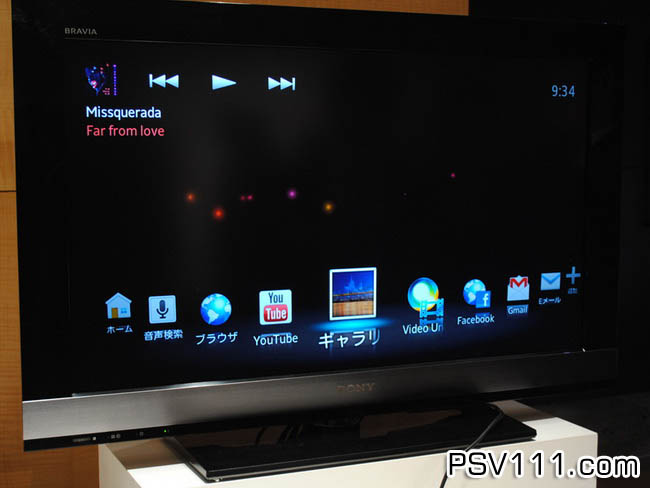The photo captures a Sony BRAVIA curved smart TV, resting on a white table against a backdrop of wood paneling. The TV, distinguished by its black screen and a silver band at the base, displaying the Sony logo, features sleek aesthetics with the "BRAVIA" logo in silver at the upper left corner. The screen is predominantly black, showing a blurred image at the center. The upper left corner includes playback controls—rewind, play, and fast-forward icons—next to the text "MISQUERADA," and beneath that, in red, "Far From Love." The time displayed on the upper right corner reads 9:34. Along the bottom of the screen are a series of nine application icons: a home icon, a microphone, a globe, the YouTube logo, a blue and orange square resembling a city skyline, a video icon, the Facebook logo, the Gmail icon, an envelope, and a plus sign. The bottom right-hand corner displays "PSV111.COM." The TV’s base is black and occupies most of the table’s width, adding to the modern and sophisticated look of the setup.

This detailed description amalgamates the shared elements and specific details provided in the original captions to offer a comprehensive view of the scene.